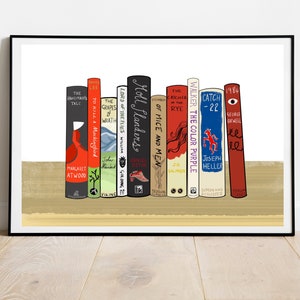This photograph, taken indoors, features a detailed painting encased in a slim black frame with a narrow grey mat. Positioned against a white wall and above light wooden flooring, the central artwork depicts a row of upright books on a light wooden shelf or table against a white backdrop. The spines of the books, some identifiable and others not, showcase solid colors and distinct titles such as "1984" (predominantly red), "Catch-22" (blue with red and white text), "The Color Purple" (white with blue text), "Of Mice and Men," and others. There are approximately eight or nine books in total, painted to mimic hardcover versions with various striking colors, including red, yellow, black, and green. The meticulous arrangement and vibrant hues suggest it may be a handmade or even a computer-generated piece of art.